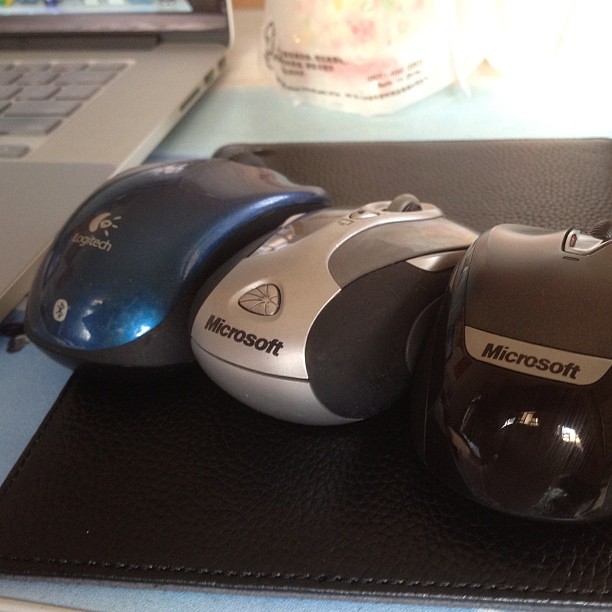This detailed photograph captures a close-up of a desk's top-left area. Dominating the upper left-hand corner, an open, silver laptop – potentially a MacBook – reveals parts of its screen and faintly visible apps. To its right lies a piece of paper with some obscure writing towards the bottom, exhibiting white and red colors. The bottom right-hand corner showcases a black leather-like mouse pad, distinguished by its neat stitching. On top of this pad are three computer mice, each placed horizontally in a row. The first is a striking blue Logitech mouse featuring its logo and a Bluetooth symbol. The middle one is a sleek black and silver Microsoft mouse, while the last mouse, also from Microsoft, is predominantly black with a silver band. A reflection in the bottom right corner of this mouse hints at a lit window nearby. This assortment of mice suggests an evolution of designs over time.